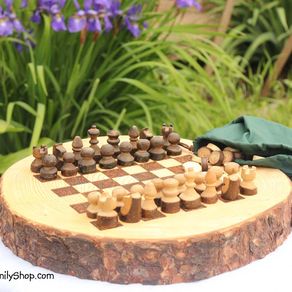In the image, a round, two-inch thick wooden log slice has been transformed into a charming chessboard, featuring alternating beige and dark brown squares. Set up for a game, the classic chess pieces are arranged with light beige pieces on the closer side and dark brown pieces on the far side. The surface of the log slice has a slight bright yellow tint around the edges, which transitions into a rich brown perimeter. Behind the chessboard, a background of long, vibrant green grasses is adorned with delicate light-purple flowers, adding a touch of natural beauty to the scene. A watermark reading "nilyshop.com" is visible in the bottom left corner, slightly overlaying the image.